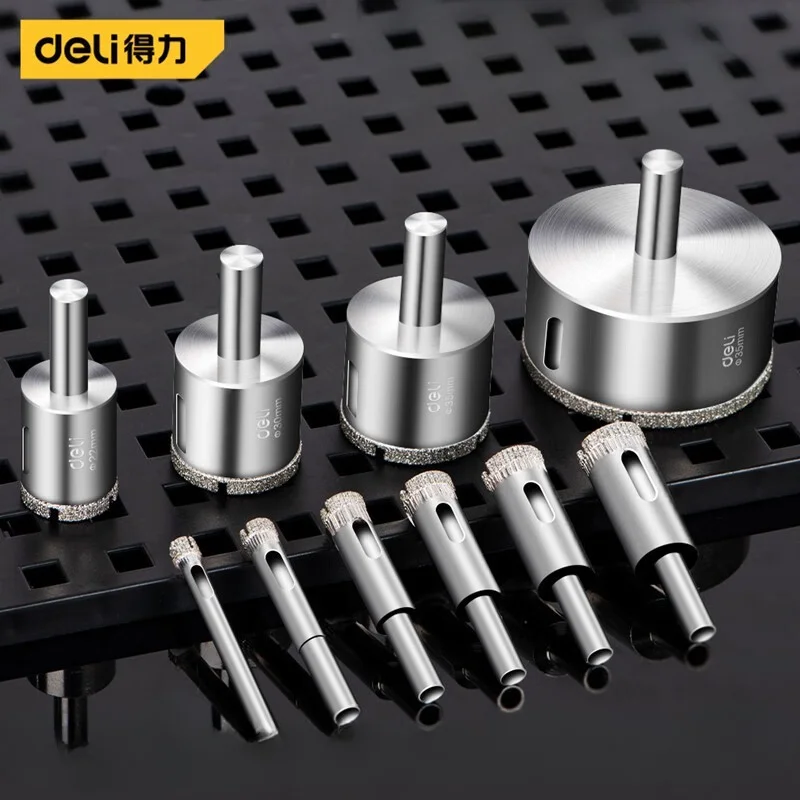The image showcases a set of brand new stainless steel tools arranged on a light black platform with evenly aligned tiny vertical squares. There are four circular tools with central rods, lined up from smallest to largest, ranging from approximately 0.22 mm to 0.35 mm in diameter. Below them are six progressively larger steel rods, starting from the smallest and stair-stepping up in size. The tools appear well-made and are likely used in a commercial setting. In the top left corner, a label reads "Deli" followed by two Chinese characters, all set against a yellow background. The precise arrangement and the pristine condition of the tools suggest they have just been manufactured and are ready for assembly.